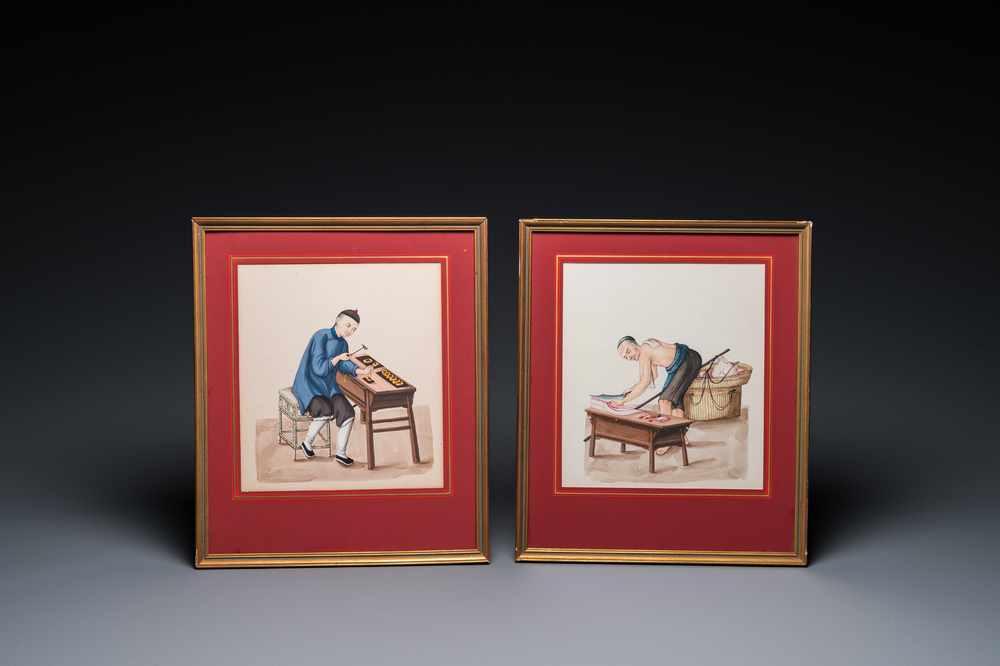This horizontally aligned rectangular image showcases two pictures framed with dark gold trim and bordered by dark red. The background transitions gradually from light gray at the bottom to dark gray at the top. Each picture features a man engaged in different activities. 

In the left frame, which has a beige center, a man donning a blue shirt and brown shorts is seated at a workbench. He appears to be using a hammer or mallet, although the specific details of his task are unclear. The workbench has four legs. 

In the right frame, the same man, now shirtless and wearing gray shorts, is shown bending over the same workbench. The nature of his activity remains ambiguous, but it involves him using some kind of tool or object. The entire scene is set against a solid black background at the top, enhancing the contrasting elements in the images and frames.